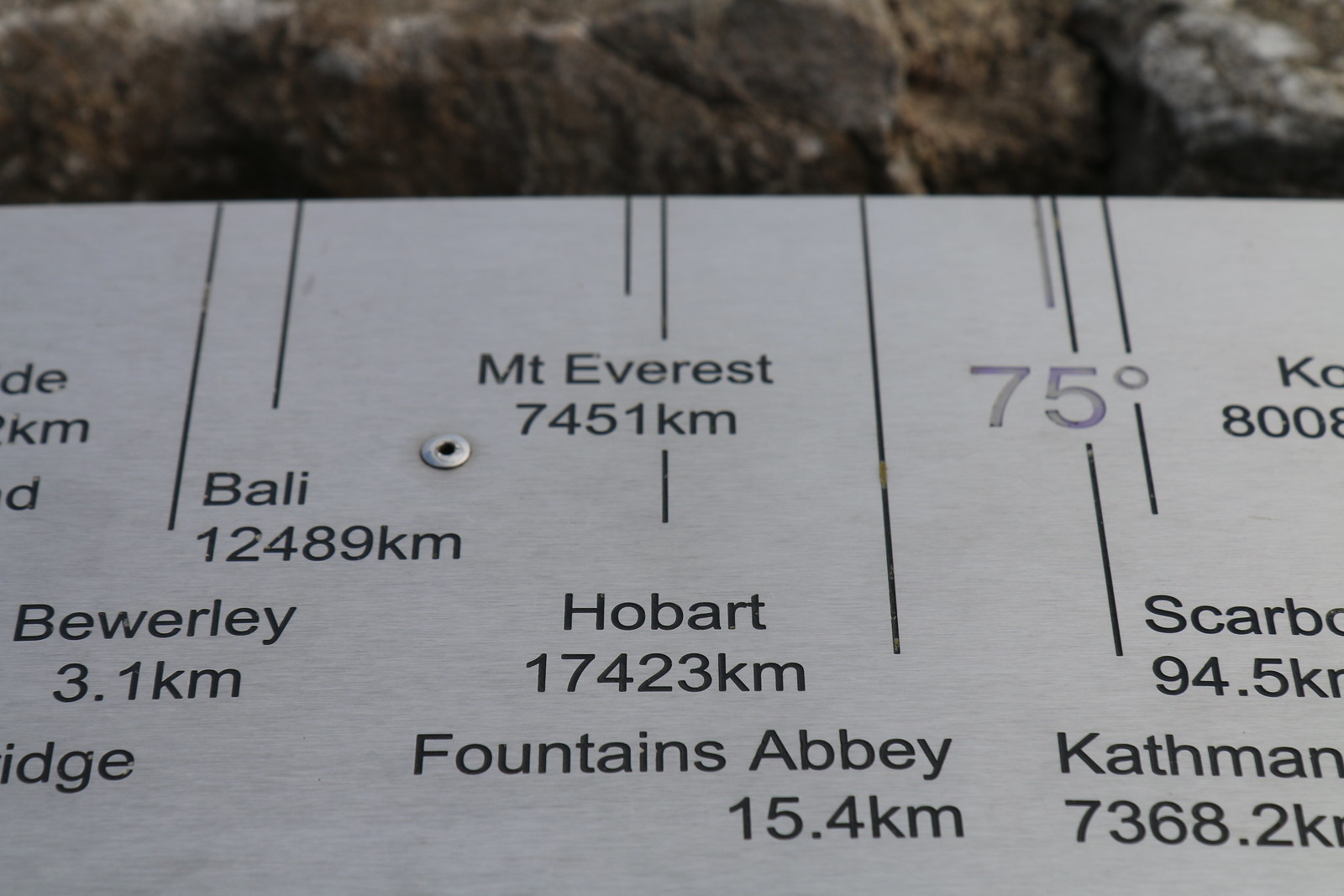This close-up photograph features a metallic, silver-colored plate with text imprinted on it, displaying the names of various places along with their respective distances. Notable locations listed include Beverly at 3.1 km, Bali at 12,489 km, Mount Everest at 7,451 km, Hobart at 17,423 km, Fountains Abbey at 15.4 km, and Kathmandu at 7,368.2 km. Next to each place name, vertical lines indicate their distances. The plate contains additional, partly visible inscriptions and a rivet on the left side. The top portion of the image shows a background of brown and grey rock formations, providing a natural setting behind the metallic plate.